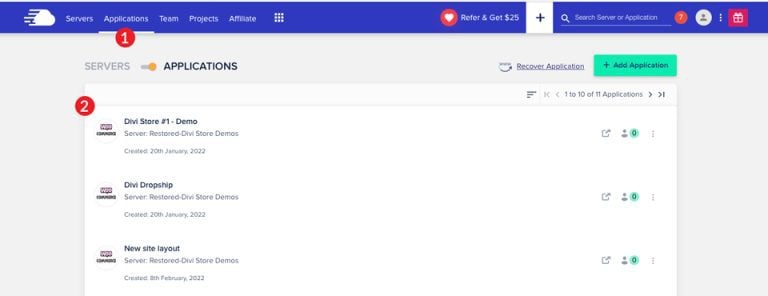Screenshot of a company's webpage designed for consumer use displayed on an office desktop. The top of the page features the company's logo. Below the logo, the navigation menu includes options labeled: Servers, Applications, Team, Projects, Affiliate. Adjacent to this menu, there's a prominent orange heart icon accompanied by the text "Refer and get $25." 

Next to this incentive, a plus sign icon is followed by a search bar for easy navigation. An orange question mark inside a circle provides help or information, and a small person icon within a circle likely indicates user account settings. Another unidentified logo is present in a separate box.

Under "Applications," there's a circular icon featuring a large orange circle with a smaller white circle inside it. Below this icon, the text "Servers" appears but is grayed out, indicating it's not currently active or selectable. Following this, there’s a narrow progress bar, and the text "Applications" is listed again. On the right-hand side, there is an option labeled "Recover Application," and a light greenish-blue button that says "Add Applications."

Beneath this section, a box marked with a number "2" in the corner contains further details. It lists "Divi Store Number One Demo," with the status "Server Restored Divi Store Demo," followed by some smaller unreadable text. Additional entries include: "Divi Dropship Server Restored Divi Store Demos" and "New Site Layout Server Restored Divi Store Demos."